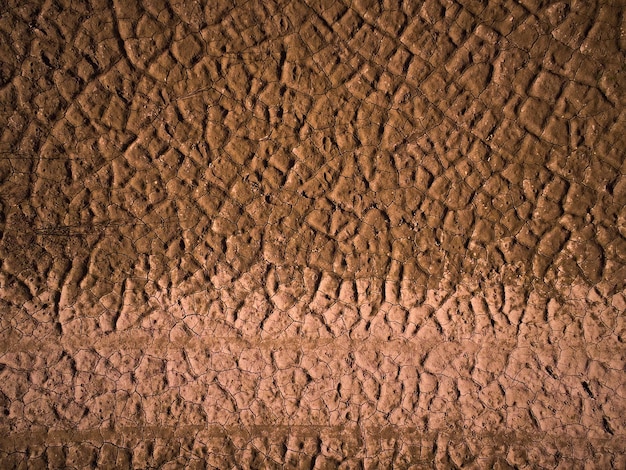The image showcases an intricate brown texture, appearing as an enigmatic and highly zoomed-in surface. Dominated by a darker brown hue in the top three-quarters and transitioning to a lighter brown at the bottom, the texture exhibits a series of grooves, ridges, and cracks. These formations resemble the complex patterns found in heavily weathered dirt, dried leather, or even a macro shot of medium-brown skin. The darker region on top displays pronounced ridges akin to the crisscrossing lines on an ice cream cone, whereas the lighter bottom third appears more flattened and blended, as if subjected to continual pressure. The absence of text further emphasizes the texture’s mysterious and visually compelling qualities.